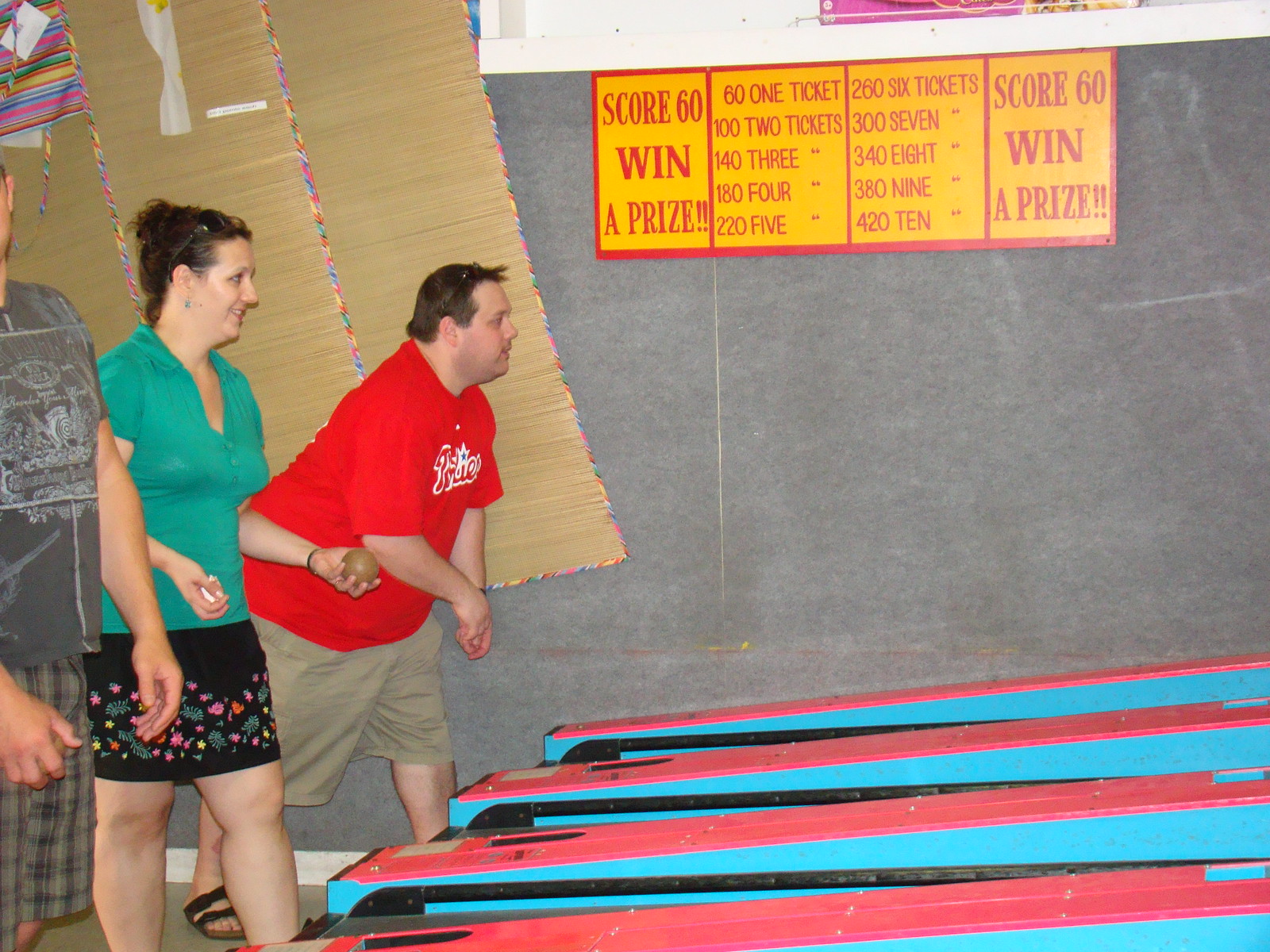The image is a horizontally aligned, rectangular frame capturing a lively arcade scene. Dominating the lower right and center of the picture are several skee-ball lanes, featuring blue sides with red tops where the balls return. In the foreground, there are three individuals engaged in the game. 

On the far right, a young man in his twenties is dressed in a red t-shirt with writing on the front, tan shorts, and brown sandals. He's bent over, appearing to have just rolled a skee-ball. Moving to the center, a woman stands poised with a brown skee-ball in her left hand, ready to throw. She sports a short-sleeved green top and a black skirt adorned with a floral pattern. Partially visible on the left edge of the frame, another man in a gray patterned t-shirt and plaid khaki shorts is captured, though only his left ear is distinguishable.

The background is dominated by a gray wall adorned with a prominent yellow and red sign displaying various ticket thresholds: "Score 60 win a prize, 61 tickets, 102 tickets, 143, 184, 225, 307, 348, 389, 420." This colorful sign punctuates the lively, competitive atmosphere of the arcade.